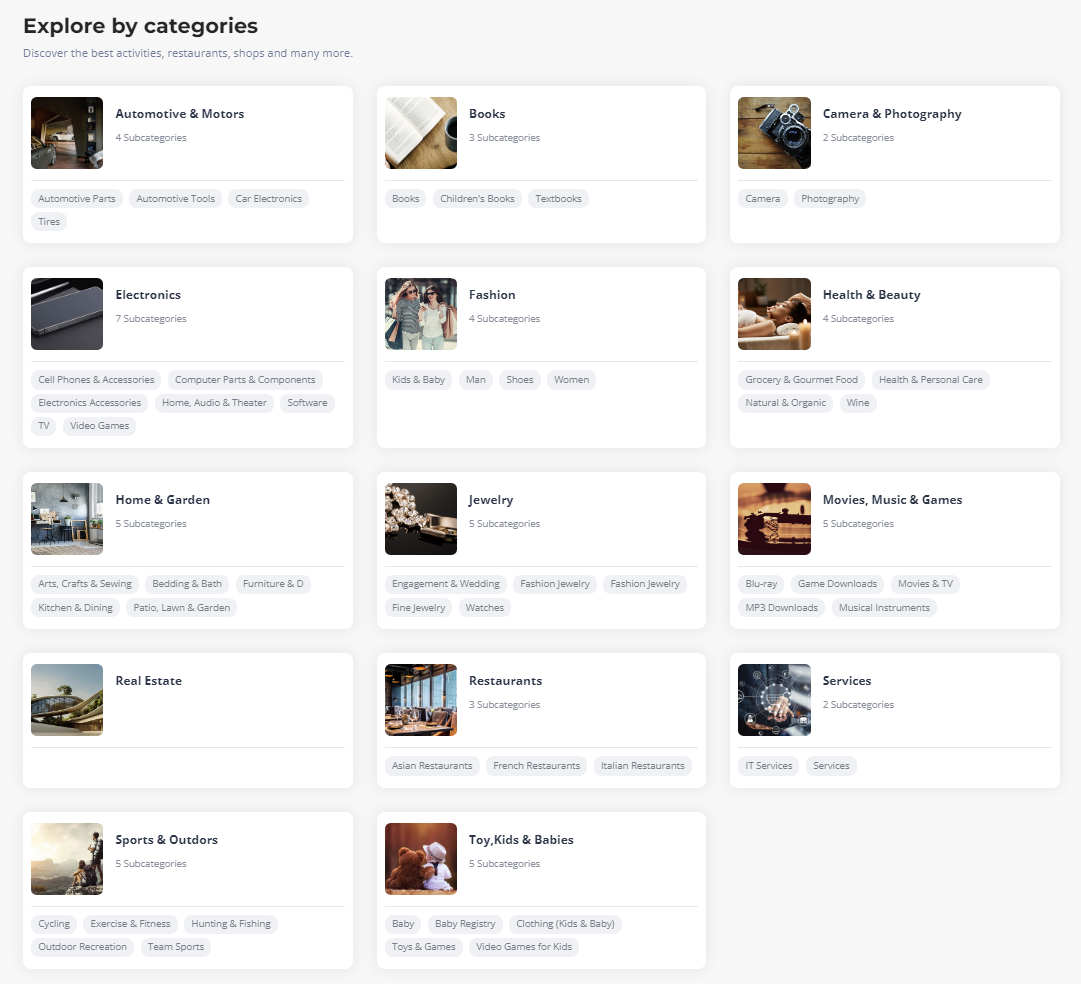The website prominently displays its purpose of serving as an advertising platform, accentuated by a navigational section in the top left labeled "Explore by Categories." This header entices users to "Discover the best activities, restaurants, shops, and many more," setting the stage for a comprehensive browsing experience.

The page layout is organized into several distinct sections composed of image-embedded rectangular blocks that symbolize various categories. The primary layout is structured as follows: three sections across the top and five sections down the page, culminating in two sections at the bottom.

Each category block features an illustrative image that represents its content:
- **Books**: Illustrated by an open book.
- **Camera and Photography**: Depicted with a camera icon.
- **Health and Beauty**: Visualized by a serene spa scene.
- **Fashion**: Showcased with two individuals donning stylish clothing.
- **Electronics**: Portrayed with an image of a laptop or mobile phone.
- **Home and Garden**: Captured by a beautifully arranged kitchen.
- **Jewelry**: Represented by a sparkling necklace.
- **Movies, Music, and Games**: Illustrated with a vinyl record spinning on a turntable.
- **Services**: Various service-related icons.
- **Restaurants**: Depicted with gourmet dishes.
- **Real Estate**: Visualized by a house image.
- **Sports and Outdoors**: Showcased by outdoor activity equipment.
- **Toys, Kids, and Babies**: Portrayed with playful toys.
- **Automotive and Motors**: Illustrated by car-related imagery.

This well-organized homepage offers users an intuitive way to discover diverse categories, each vividly represented by corresponding images, thus enhancing the search and browsing experience.